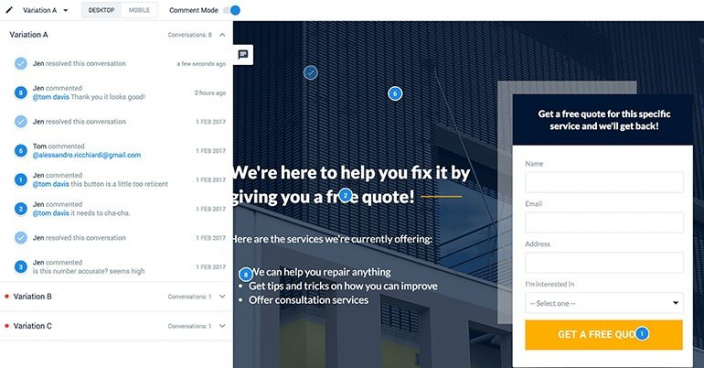The left third of the image depicts a vertical column with a white background, containing several tabs at the top labeled as "Variation A," "Desktop," "Mobile," and "Comment Mode." The title "Variation A" stands out at the top left in bold text. Below this title, a series of icons in various shades of blue are displayed, representing different user actions. While the text adjacent to these icons is too small to read, one can infer that they are similar to social media activity indicators, such as comments or timestamps. There are approximately eight to ten of these blue icons arranged vertically.

Towards the bottom of the column, distinct categories labeled as "Variation A," "Variation B," and "Variation C" appear, suggesting the ability to navigate through different sections or versions by interacting with these tabs.

In the background, occupying the right two-thirds of the image, there is a website banner. The visible portion of the banner showcases the exterior of a building, rendered in dark blue or dark gray hues. This banner contains a form on the right side prompting users to "Get a free quote for this specific service." The form fields include sections for "Name," "Email Address," "Address," among other details, facilitating user engagement.